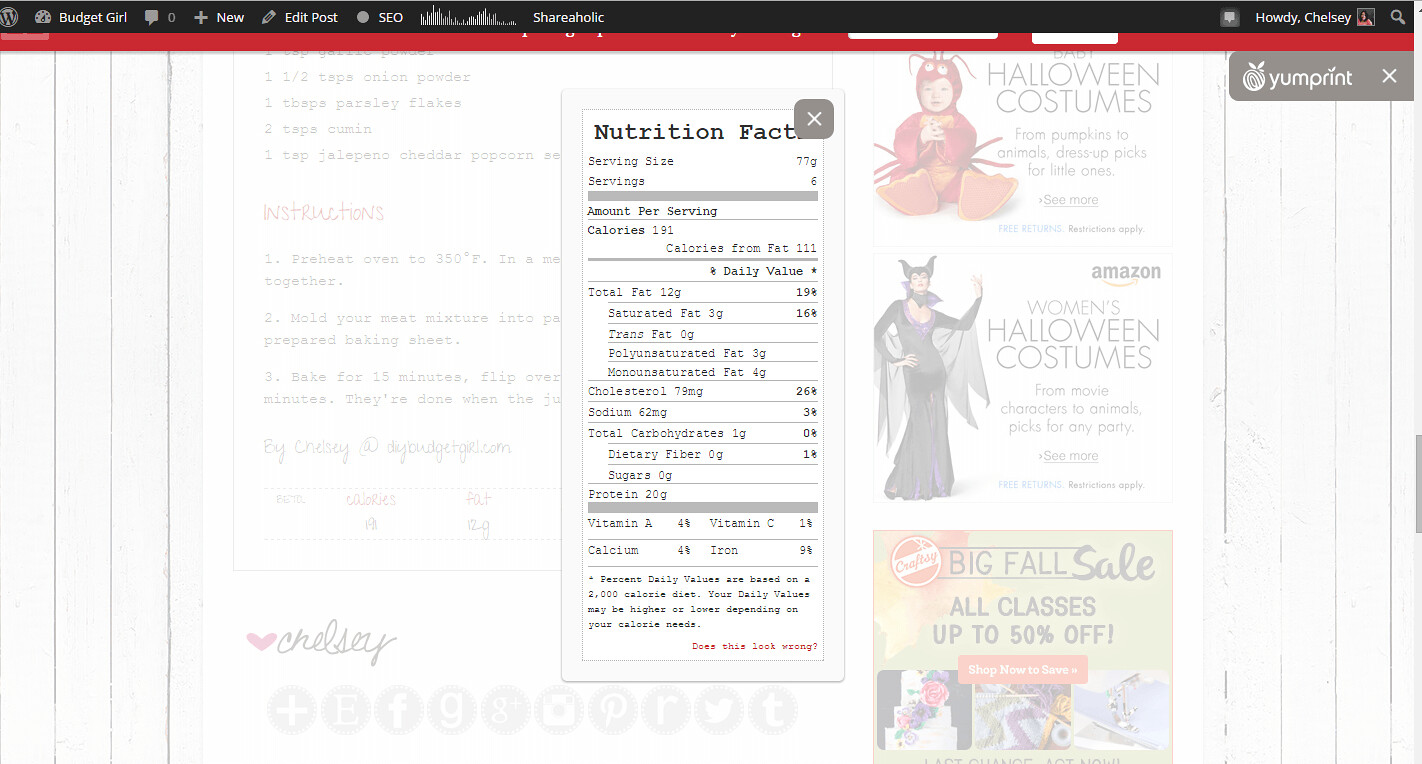This image depicts a screen capture of a profile page belonging to Chelsea Howdy on the website Yumprint. The interface is faint and pale, with Chelsea's name prominently displayed in the top right corner. On the left side of the screen, a recipe is partially visible, showing both the ingredients and instructions. The central area features a detailed nutrition facts panel, providing an in-depth look at the nutritional value of the recipe. To the right, there are a series of secondary content ads: one for women's Halloween costumes, another for children's Halloween costumes, and a prominent advertisement for a major fall sale. The layout and design elements suggest an organized, yet slightly muted, visual presentation typical of the Yumprint platform.